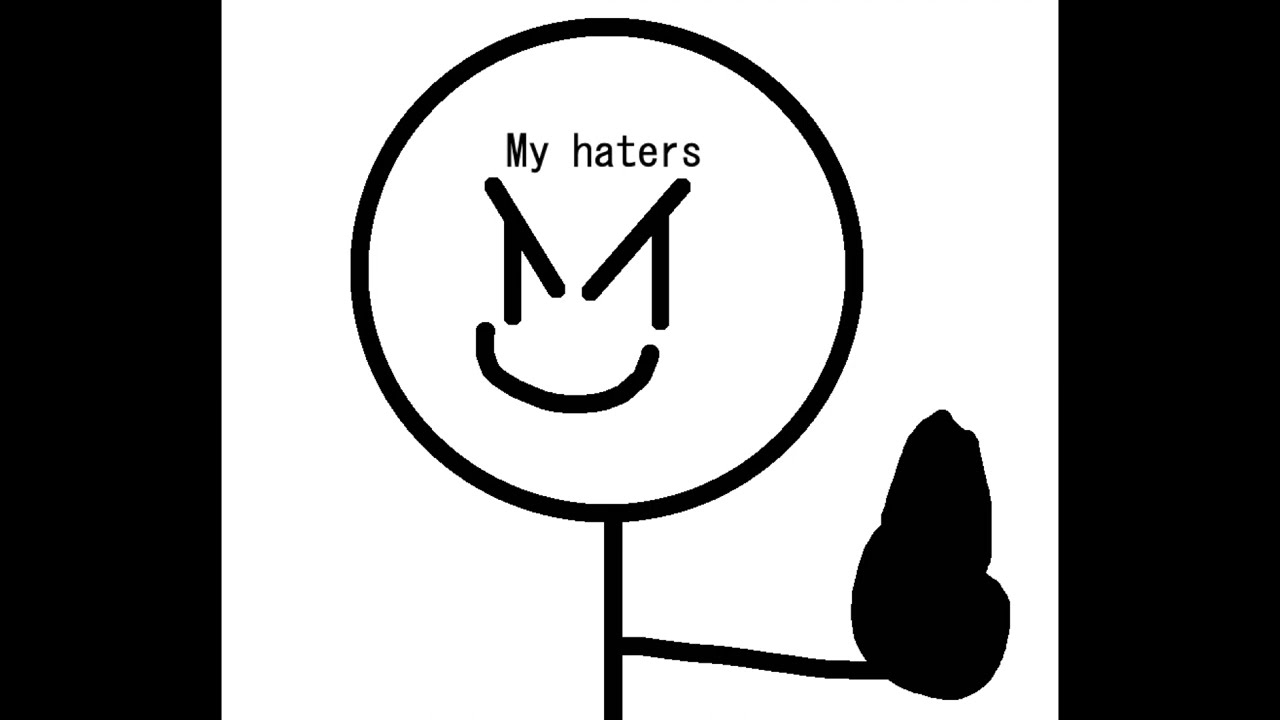The image features a computer-made stick figure drawing on a white background, framed by thick black vertical bars on either side, creating a letterbox landscape perspective. At the center of the image, there is a large, perfectly circular head occupying about a third of the frame. The character’s facial expression includes two vertical slit eyes, slanted inward, suggesting evil, slanted eyebrows. Beneath the eyes is a slightly askew smile. The text "My Haters" appears prominently in a small Courier font on the forehead of the character. The stick figure, colored entirely in black, extends its left arm outwards, holding what seems to be a black object that could be interpreted either as a hand or a gun. The lack of color variation and the simplistic design emphasize the sinister yet smug demeanor the figure conveys, potentially intended as a message to those the creator considers adversaries.